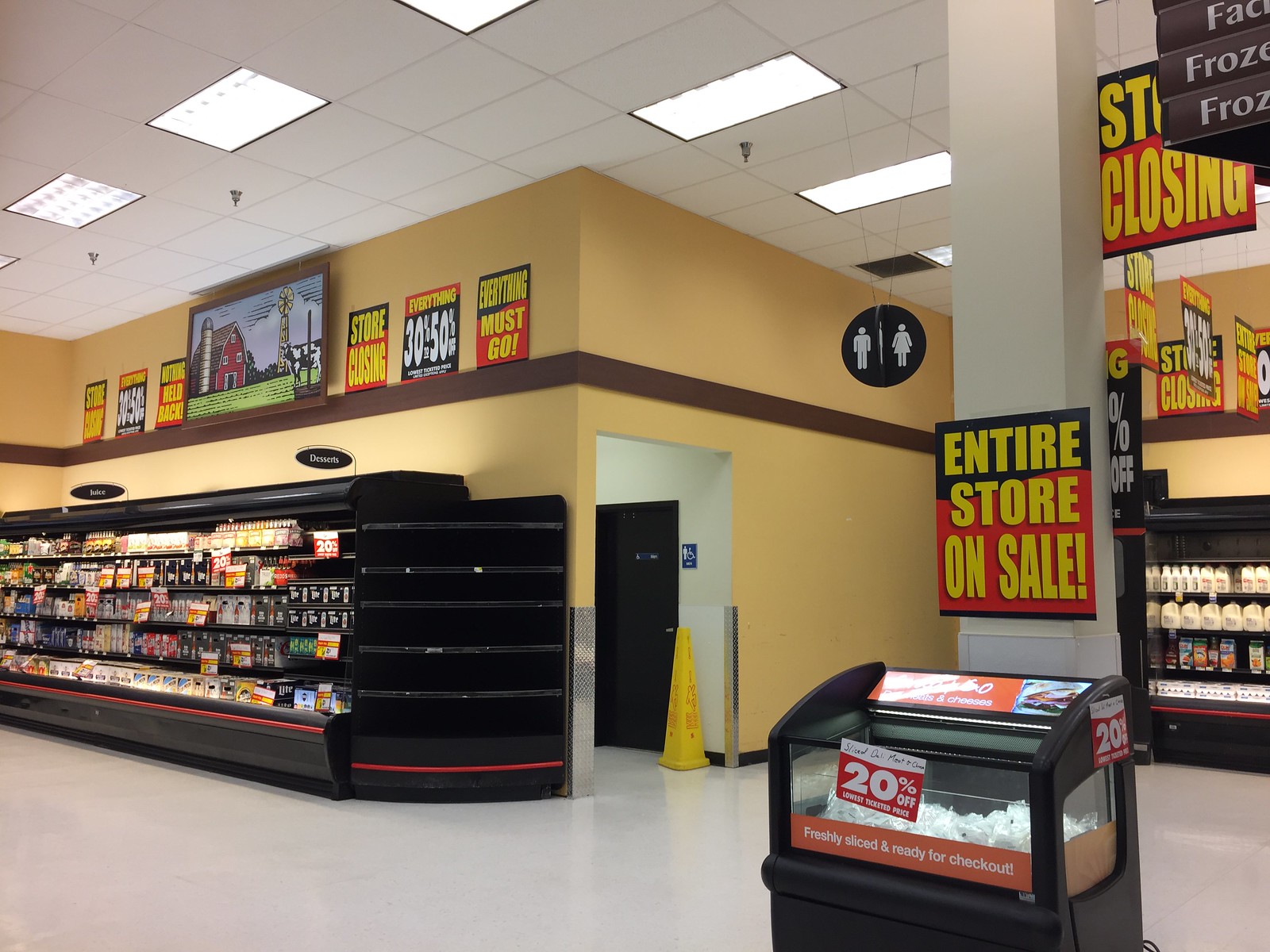The image depicts the interior of a retail store with a yellow-painted wall. The ceiling, adorned with recessed lighting, adds a bright illumination to the scene. The yellow wall extends around a corner that leads to the entrance of the bathrooms. To the left, there is a large display shelf reminiscent of a grocery store's dairy section, stocked with various yogurts and drinks. Above this shelf, there is a picture featuring a barn and silos, flanked by bold signs in black, red, and yellow proclaiming, "Store Closing. Everything Must Go. Everything 30 to 50 percent off." To the right, there is a prominent column partially obscuring the milk section. This column bears a "Store on Sale" sign. Directly in front of the column is a bin filled with white-packaged containers, marked with a sign indicating a 20% discount.